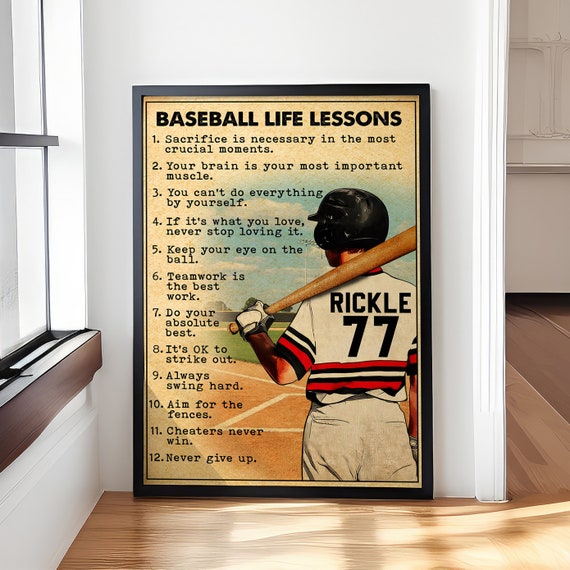The photograph captures a framed poster propped up in the corner of a room with a wooden floor and white walls, with one wall featuring a window. The poster displays "Baseball Life Lessons" in bold black text at the top, followed by twelve inspiring lessons: 1. Sacrifice is necessary in the most crucial moments. 2. Your brain is your most important muscle. 3. You can't do everything by yourself. 4. If it's what you love, never stop loving it. 5. Keep your eye on the ball. 6. Teamwork is the best work. 7. Do your absolute best. 8. It's okay to strike out. 9. Always swing hard. 10. Aim for the fences. 11. Cheaters never win. 12. Never give up. Alongside the text, a picture of a baseball player is visible to the right. The player, with his back to the camera, is in a white, red, and black uniform with the name "RICKL" and the number 77 on his jersey. He holds a bat slung over his shoulder and wears a helmet, standing on what appears to be a baseball field. The framed poster, leaning against the walls, with clear details of both the setting and the poster's content, gives off a vintage vibe and captures the essence of passion for baseball.